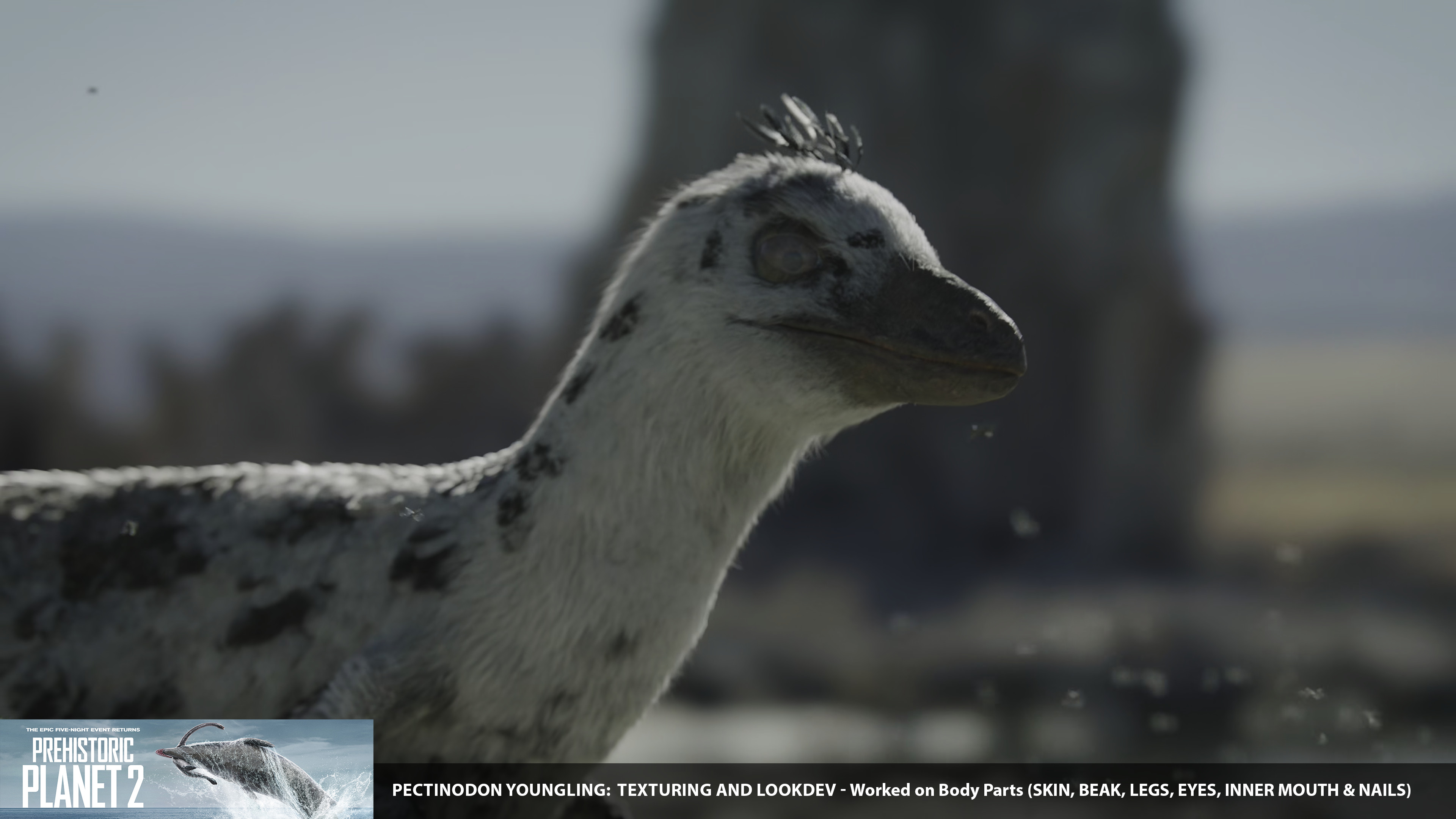The image depicts a pectinodon youngling, showcased as part of an advertisement for a television program titled "Prehistoric Planet 2," indicated by text at the bottom left of the image. The creature resembles a bird but with a much thicker body and neck. Its skin has a distinctive pattern, featuring white fur with black leopard-like spots extending from the eyes to the back, reminiscent of a Dalmatian's coat. The youngling has a round head adorned with black tufts of feathers, a thick black beak, and gray eyes that blend with its fur. Only the upper part of its four-legged body is visible against a blurred natural background with elements like large rocks, plain land, and some bushes. The caption also highlights various texturing and look development efforts on its body parts, including the skin, beak, legs, eyes, inner mouth, and nails. The size of the pectinodon is comparable to that of a golden retriever.